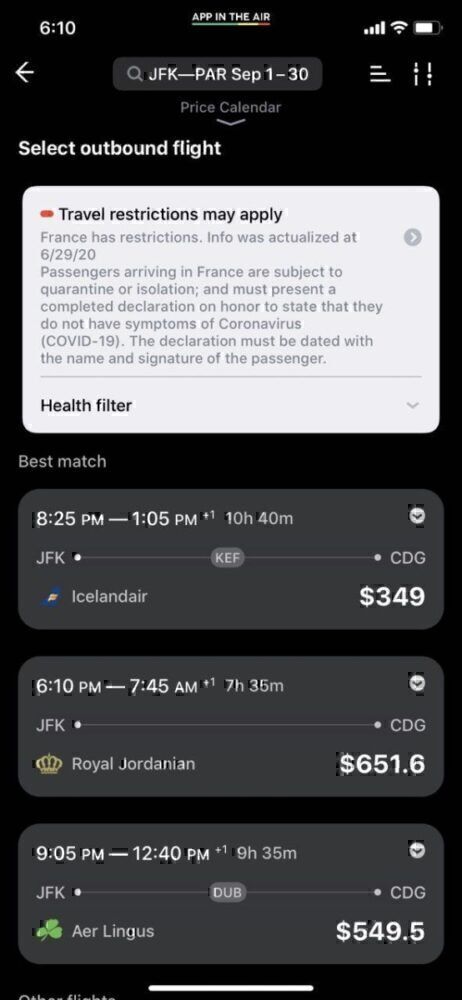The image features a screenshot of a flight booking app called "App in the Air." At the top center, it lists flight details: JFK to PAR (Paris) for travel between September 1 and 30. Below this, there is a dropdown labeled "Price Calendar." 

To the left, there is a prompt titled "Select Outbound Flight." A disclaimer notes that "Travel restrictions may apply," specifically stating that France has restrictions that were last updated on June 29. It mentions that passengers arriving in France are subject to quarantine or isolation. They must also present a completed declaration, signed and dated, asserting they do not have COVID-19 symptoms.

Underneath, there is a section labeled "Health Filter," followed by a "Best Match" for flights from JFK to CDG (Charles de Gaulle Airport in Paris). The options listed include:
1. Iceland Air for $349.
2. Royal Jordanian for $651.
3. Aer Lingus for $549. 

Each option showcases different prices and airlines available for the specified route.